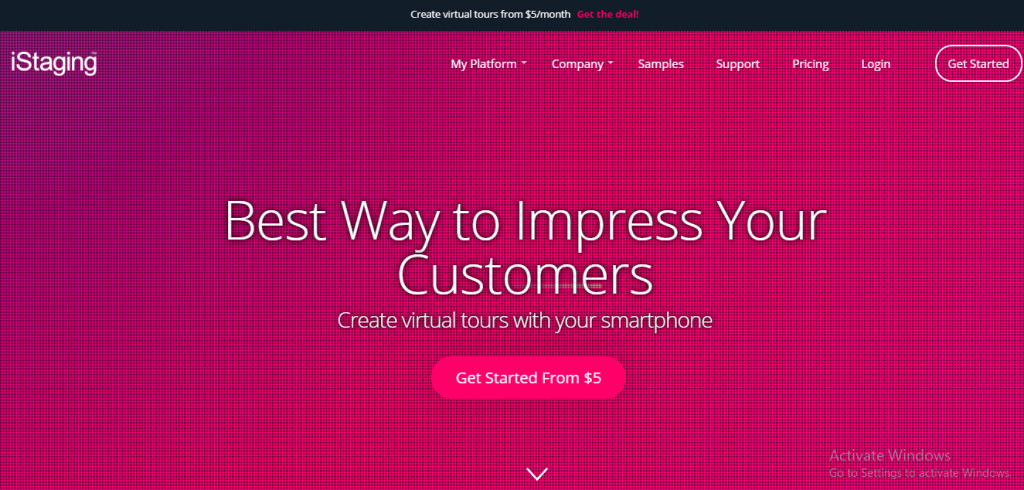This web page features a prominent maroon red section dominating most of the screen, complemented by a thin, dark black bezel lining the top. Centered in this maroon section is a bold headline in white text reading, "Create virtual tours from $5 a month." On the right-hand side of this headline, there is a vibrant hot pink call-to-action button with the text, "Get the deal!" and an enthusiastic exclamation mark.

To the left of the maroon red area, the brand name "iStaging" is displayed in bold white lowercase letters. Adjacent to the right, there is a horizontal navigation menu with multiple clickable buttons. The first button, labeled "My Platform," features a downward-facing white arrow, indicating a dropdown menu. Following this are buttons labeled "Company," "Samples," "Support," "Pricing," and "Login." 

On the far right side, there is an oval button with a white border and internal white text that reads, "Get Started." 

Dominating the central area of the web page is a bold white statement, "Best way to impress your customers," with a subtext in gray indicating, "Create virtual tours with your smartphone." Beneath this, another call-to-action oval button in hot pink with white text states, "Get started from $5."

At the very bottom of the maroon red section, a downward-pointing arrow in bold white hints that more content is available below, encouraging users to scroll down. To the right, there is a semi-transparent gray text notification from the operating system that reads, "Activate Windows - Go to Settings to activate Windows."